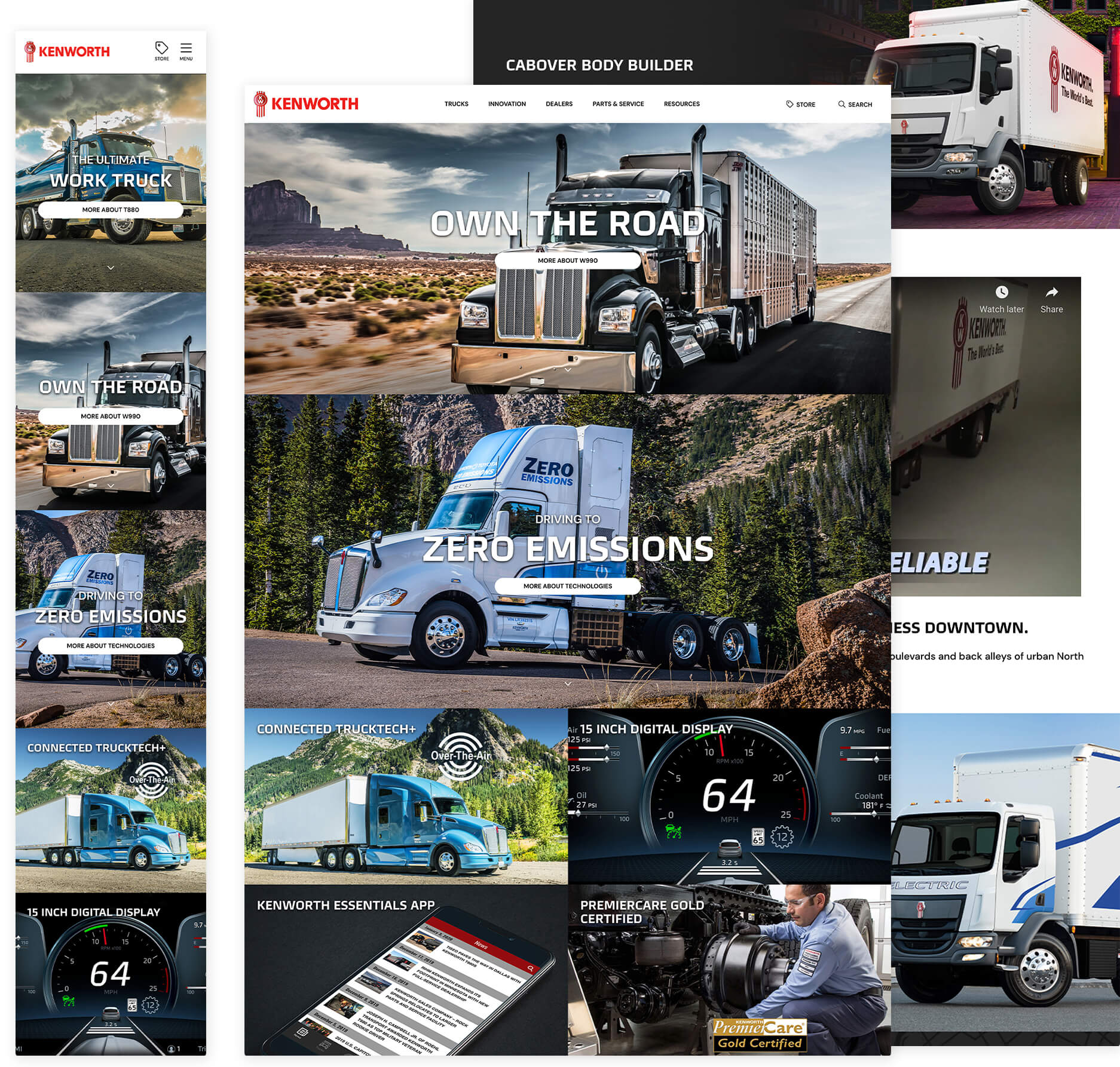This detailed caption provides a comprehensive description of a screenshot from Kenworth’s official website, outlining its layout and visual elements:

---

This screenshot captures Kenworth's official website interface. At the top left corner, the Kenworth logo and the brand name "Kenworth" in red capital letters are prominently displayed. Below these, there's a tag labeled "Store" next to a hamburger menu icon. This section is positioned above a vertical stack of images on the left-hand side.

1. **Top Image**: The image showcases a blue Kenworth T-880 truck with a gas tank mounted on its rear, captioned "The Ultimate Work Truck." A link for more information about the T-880 is provided.
2. **Second Image**: This displays a sleek black Kenworth W-990 truck, an 18-wheeler hauling a large box trailer. The caption reads "Own the Road" with additional details about the W-990.
3. **Third Image**: A white truck with blue accents and the words "Zero Emissions" is featured against a backdrop of evergreen trees and mountains. The caption highlights Kenworth's commitment to zero emissions, with a link for more information about their technologies.
4. **Fifth Image**: Highlights "Connected Truck Tech Plus," featuring a light blue Kenworth truck with a white trailer, and an overlaid graphic of three concentric circles with the text "Over the Air" running through them. Mountains provide a scenic background.
5. **Sixth Image**: Shows a 15-inch digital display with the speedometer reading "64," complemented by a steering column ascending from the bottom.

The middle and right sections of the page are described as follows:

- A white flat-fronted truck labeled "Cabover Body Builder" is presented in a horizontal rectangle spanning from slightly before halfway to the far right of the screen. Part of the truck's cab is obscured by this main content block. The truck is underscored by the phrase "Kenworth, the world's best."
- Remaining visible sections list menu items such as "Trucks, Innovation, Dealers, Parts and Service, and Resources," alongside the "Store" and "Search" options.

Additional images and sections on the main content area include:

- A black truck, captioned "Own the Road," appears to be a cattle carrier traversing a desert landscape with mountain formations and sparse vegetation in view. 
- A repeated "Zero Emissions" truck with evergreen and mountainous scenery.
- Another image of the "Connected Truck Tech Plus" showcasing the same blue truck with a circular "over-the-air" graphic against a mountain backdrop.
- An illustration of a 15-inch digital display, reiterating the speedometer at 64 mph.
- The "Kenworth Essentials" app depicted on a smartphone screen against a black background.
- "Premier Care Gold Certified" illustrates a technician working on a truck wheel hub, emphasizing Kenworth’s premium maintenance service.

To the right of the main webpage block, partial imagery includes:

- Part of the word "reliable" sticking out next to a partially visible Kenworth truck.
- Top indications, such as "Watch Later" or "Share."
- "S-Downtown" emerging from underneath the block, extending to "boulevards and back alleys of Urban North."
- An additional image showcasing a white and blue flat-front truck labeled "Electric" with cargo in the back.

---

This detailed caption provides a thorough overview of the visual and textual content present within the Kenworth website screenshot.